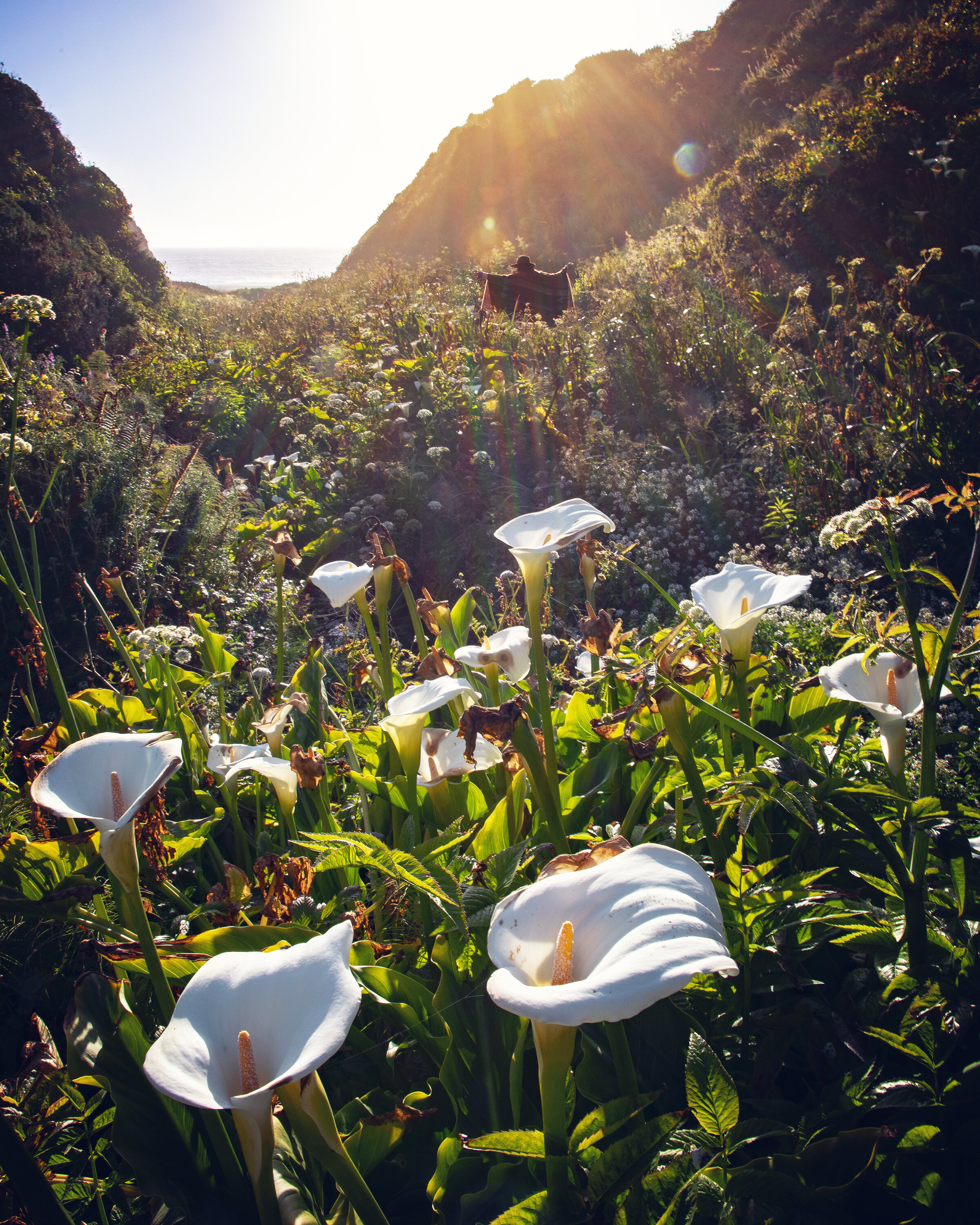The photograph captures a picturesque field abundantly dotted with vivid white flowers, primarily concentrated towards the foreground. These delicate blooms, characterized by a white opening with a long petal on one end and a shorter one on the other, display a distinctive yellow center reminiscent of corn on the cob. Interspersed among the flowers are green leaves and occasional brown leaves. Beyond this dense floral array, more of these flowers stretch back, albeit sparsely, to the left of the center of the image, fading into the distance. 

Dominating the background, a solitary figure stands silhouetted against the bright sunlight. This person, clad in a brimmed hat and a flowing robe or multicolored poncho in hues of red, green, and pink, holds their arms outstretched, creating dramatic folds of fabric that dip down. The landscape around them features a large, grass-covered hill extending to the right and a slightly smaller one to the left, between which a sliver of gray ocean is visible. While the foreground is sharply focused on the white blossoms, the distant hills and sky—painted in gradients of blue and white—augment the serene, natural ambiance of the scene.